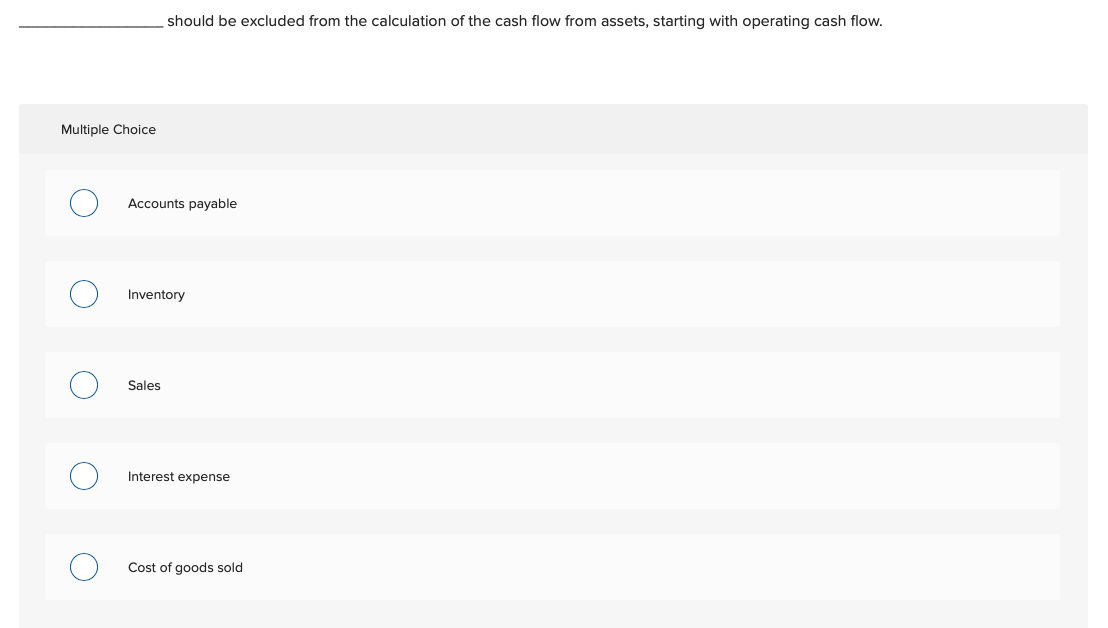The image depicts a very plain, nondescript web page interface. The background features a subtle light gray gradient with a gray box centrally positioned. Within this gray box are five elongated white text fields arranged vertically, each labeled with black text: "Accounts Payable," "Inventory," "Sales," "Interest Expense," and "Cost of Goods Sold." Each of these labels has an accompanying circle to its left, intended as selectable options, though none are currently selected.

At the top of the gray box, in prominent black lettering, is the title "Multiple Choice," though no further instructions or context are provided. The design is stark and minimalist, with no additional information about the origin, purpose, or authorship of the content. There are no company logos, contact details, or footer to offer clues about its source. The interface's simplicity and lack of distinguishing elements make it unclear whether it is meant for a desktop computer, a mobile device, or another platform. The website appears as a generic form, void of interactiveness or detailed guidance.